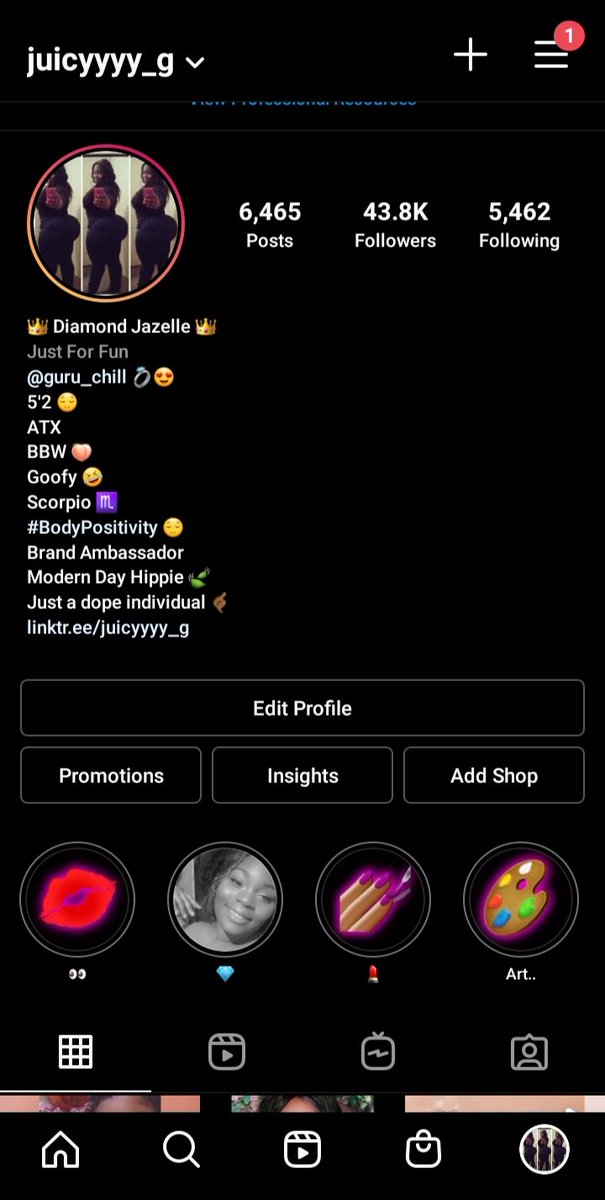The image portrays a vibrant and detailed Instagram profile. In the top left corner, the username is displayed as "Juicy" with an extended spelling using four 'Y's. To the right of the username is a white plus symbol and a hamburger menu icon adorned with a red notification circle. Below this is a colorful circular profile picture featuring three women standing and looking into a mirror.

The profile statistics show that there are 6,465 posts, 43.8 thousand followers, and 5,462 following. The profile includes several icons and text elements like a crown, Texas icon, diamond, and the name "Gizelle" placed on the crown. Additional descriptors include "Great Texas," "Just for fun," and the handle "@glue_chill." Further emojis and descriptors listed are a ring, heart eyes, Texas, "ATX," "BBW," "Goofy," "Scorpio," "Body positivity," "Brand ambassador," "Modern day hippie," and "Just a dope individual." A link to "linktr.ee/juicy" is also included. The background color of this section is black.

The profile interface shows options such as "Edit Profile," "Promotions," "Insights," and "Shops." There are various imagery elements like a pair of painted nails, a makeup palette, and a grid feed layout. Navigation icons at the bottom are depicted as a house (home button) and a magnifying glass (search function).